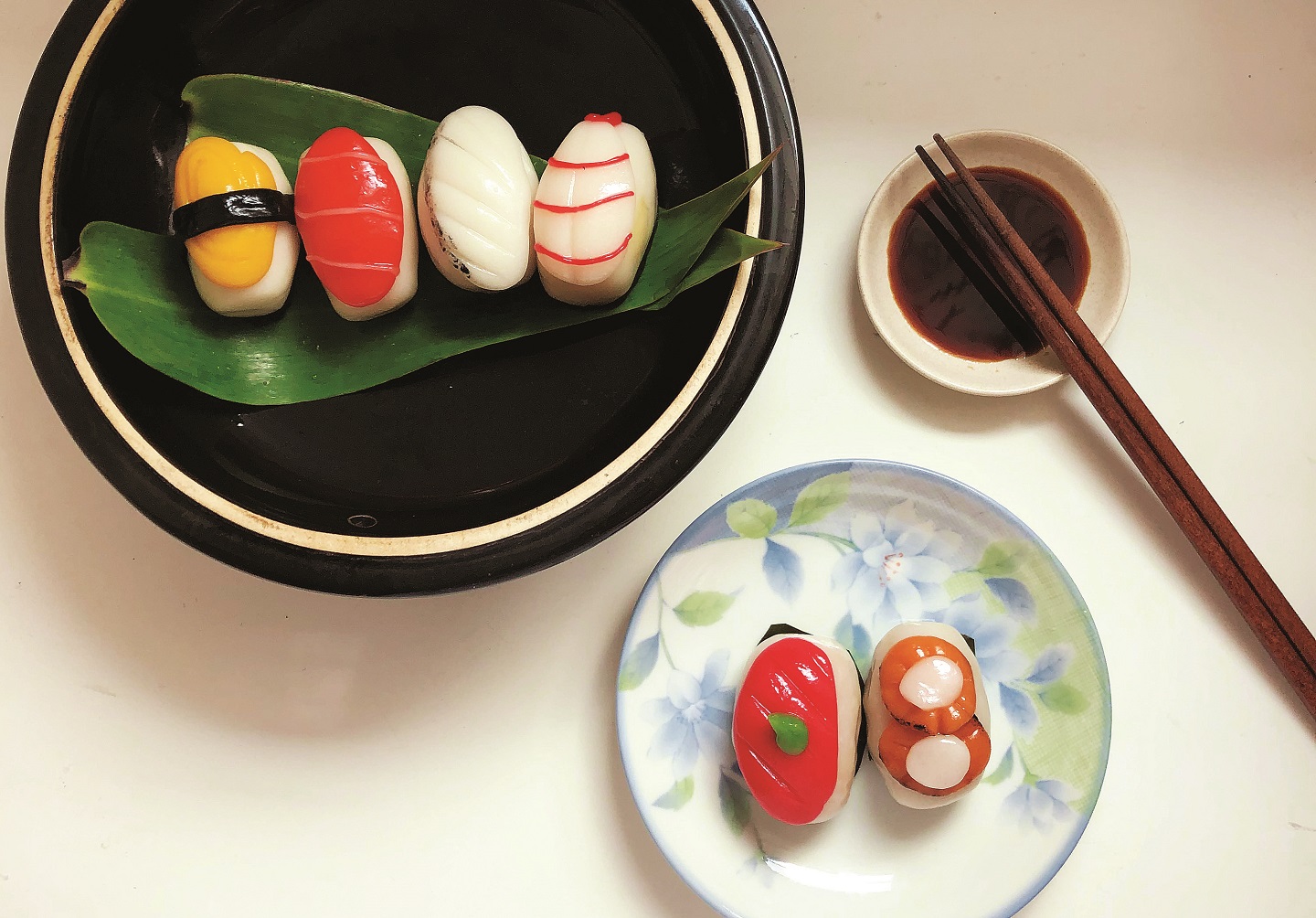The image depicts an artfully arranged lunch, featuring a varied assortment of sushi displayed on a pristine white table. In the upper left, a dark green plate with a white rim is adorned with two bamboo leaves. Resting on these leaves are four sushi pieces: one with a pinkish-red fish, one with a white fish accented with red stripes, another white piece topped with a yellow area and secured with a black band, and a final piece of white fish with a red sauce streak. 

Directly below, a floral china plate decorated with purple flowers and green leaves holds two more sushi items. One piece features seaweed, rice, and a minute dot of wasabi, while the other has seaweed, rice, and fish with a small white topping. 

Above this plate, a small saucer filled with soy sauce is present, with a pair of dark brown chopsticks resting on top and extending onto the table. The arrangement is visually striking, likely invoking the high standards of food photography for magazines or social media.